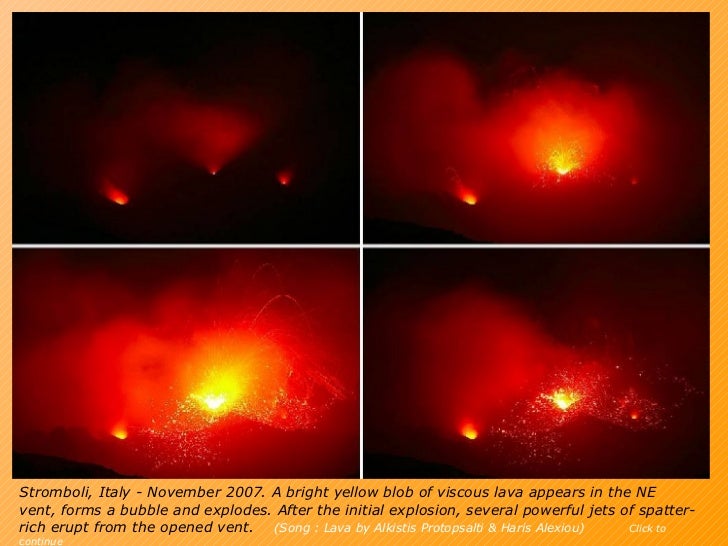This captivating image collage from Stromboli, Italy, taken in November 2007, documents the explosive activity of an active volcano in a series of four distinct phases. The composite comprises two photos on the top row and two on the bottom. Each of these frames captures a progressive stage of the volcanic eruption. 

In the initial frame, we glimpse a delicate, glowing spot of magma beneath a subtle steam cloud. Moving to the second frame, the activity intensifies as the lava starts to erupt, accompanied by a larger glow and more steam. The third frame presents the zenith of eruption, with a brilliant yellow core at the center, surrounded by red-hot lava and thick smoke, portraying the chaotic vigor of the eruption. Lastly, the final frame depicts the scene's aftermath, where the eruption begins to subside. The dispersing smoke reveals the cooling, red magma interspersed with yellow patches from the core.

The descriptive text at the bottom states, "Stromboli, Italy, November 2007," and goes on to narrate the dynamic process: a bright yellow blob of viscous lava appearing in the northeast vent, forming a bubble, and then explosively bursting. Following this initial explosion, several powerful jets of splatter-rich lava erupt from the now-open vent, vividly captured throughout the series.